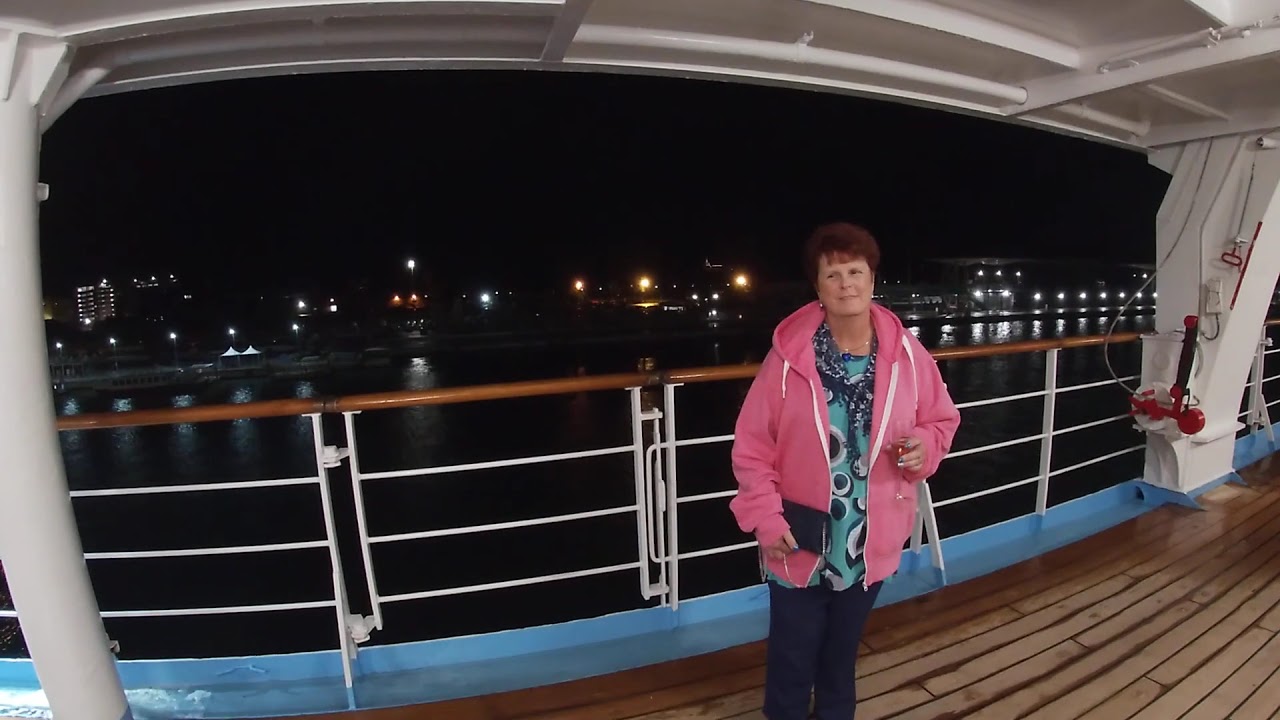In this nighttime photograph, an older woman with short red hair stands on the wooden deck of a cruise ship. She is wearing a distinctive pink jacket with white straps over a teal and blue floral top and dark blue jeans. The woman holds a beverage in her left hand and a small dark-colored purse. Her outfit is complemented by a blue and white scarf. She stands beside a white steel railing topped with a brown wooden bar. The dark sky above contrasts with the distant cityscape, dotted with bright lights from buildings and light poles. Wires and an indistinct red object are visible to the right of the image. The woman gazes towards the camera, framed by a serene aquatic backdrop and the sturdy metal structure of the ship.